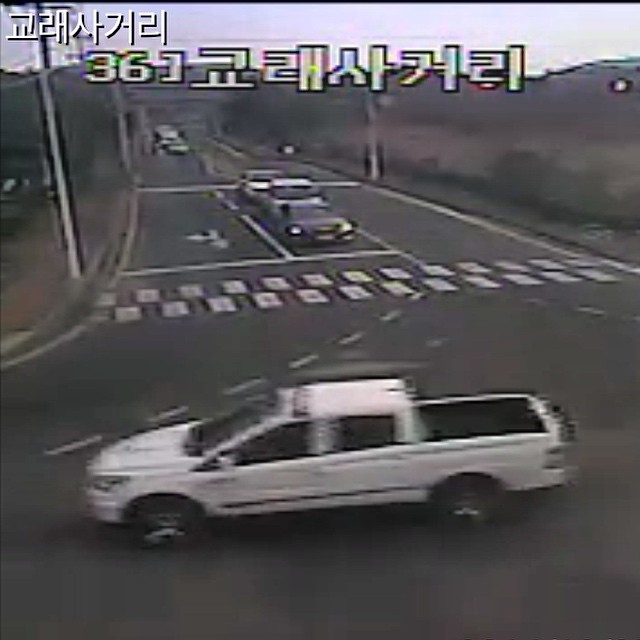A black and white photograph, seemingly captured by a traffic camera in Japan, showcases a bustling intersection. In the foreground, at the bottom of the image, a horizontal roadway intersects with a three-lane road that extends diagonally, slightly to the left as it recedes into the distance toward the top of the image. At the intersection, a white pickup truck is traversing from right to left. Adjacent to the pickup truck, a couple of cars wait in the left-turn lane, indicating their intention to turn to the right side of the image. Further back, approximately a block away, a queue of vehicles occupies the straight-ahead and right-turn lane, patiently waiting their turn.

Flanking either side of the roadway, patches of dried brush and low-lying bushes break up the landscape. The horizon in the background is uneven, marked by low-level hills or a tree-lined area, creating a rugged backdrop. In the top left of the image, Japanese characters are visible in white, though they might alternatively be Arabic. Dominating the center-right area across the tree line, a lengthy series of yellow numbers is prominently displayed, adding an element of numerical detail to the scene.